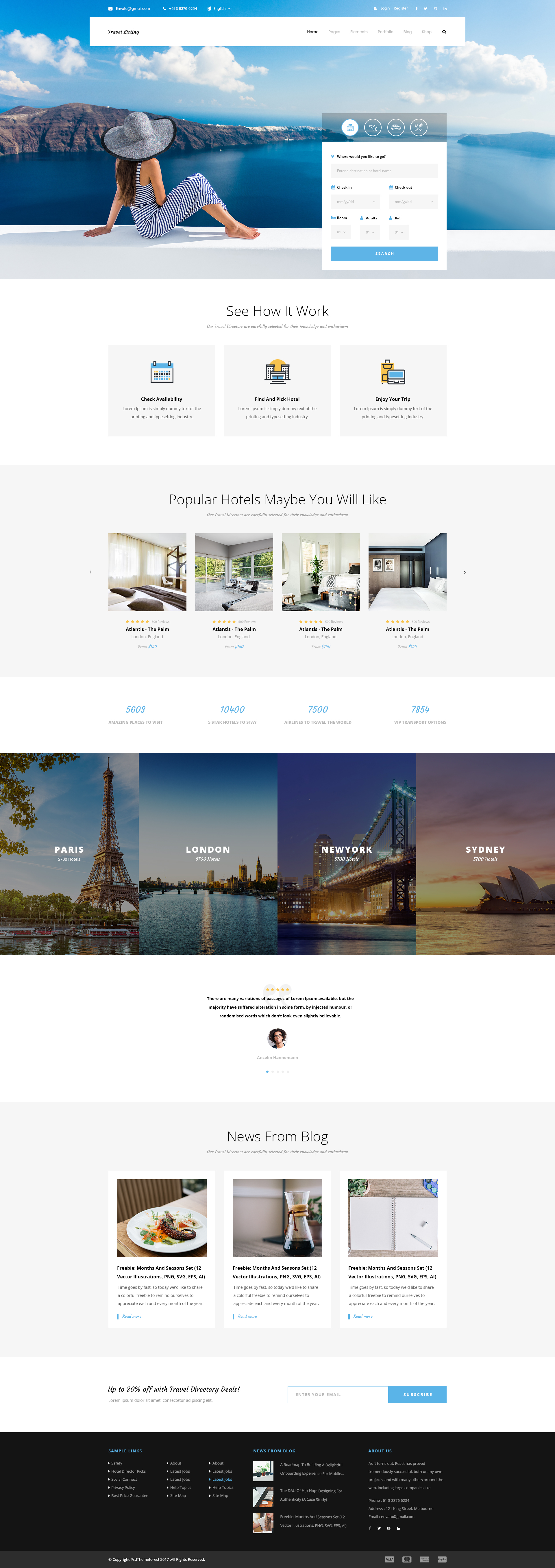A screenshot of a travel-related website displayed on a desktop. The image includes the entire website page, making the text difficult to read. 

At the top of the page, there is a prominently featured search bar next to a picture of a woman relaxing and gazing over a stunning ocean and mountain landscape. To the right of the image are search options.

Directly below this, the content shifts to a white background with a typical advertising layout. There are three squares providing an explanation under the heading "See How it Works."

Further down, a section titled "Popular Hotels You Might Like" displays four hotel options, each accompanied by a picture.

Following this, the website showcases four major cities, each represented with an image: Paris, London, New York, and Sydney.

At the bottom of the page, there is a segment titled "News from the Blog," likely featuring the latest articles or updates.